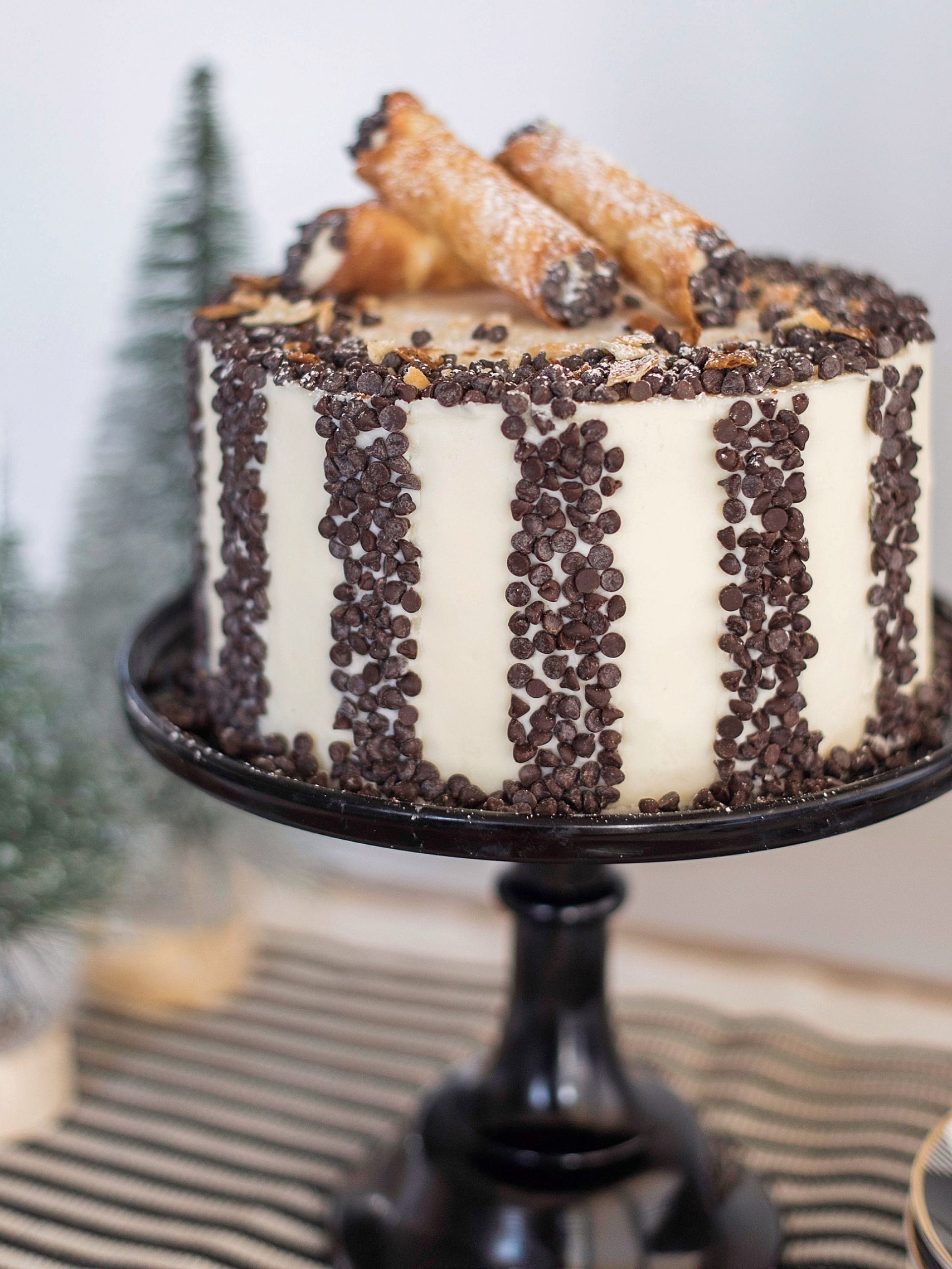This high-definition food blog photograph showcases an elegantly decorated dessert cake, artfully presented on a dark brown ceramic stand with a tapered neck and broad base. The cake, possibly a tiramisu or a white cream cake, features beige icing with a design of milk chocolate drops spaced an inch apart, cascading from the top to the bottom of the cake and spilling slightly onto the stand. The top is embellished with an outer ring of these chocolate drops and three crunchy cannoli rolls filled with cream and dusted with powdered sugar, their ends also adorned with chocolate drops.

In the softly blurred background, adding a festive touch, are two small ornamental green trees on a tan and black striped table mat, placed on a table next to a wall. The scene is set for a holiday or special occasion, with the primary focus being the beautifully detailed cake that takes center stage in this captivating and mouth-watering image.